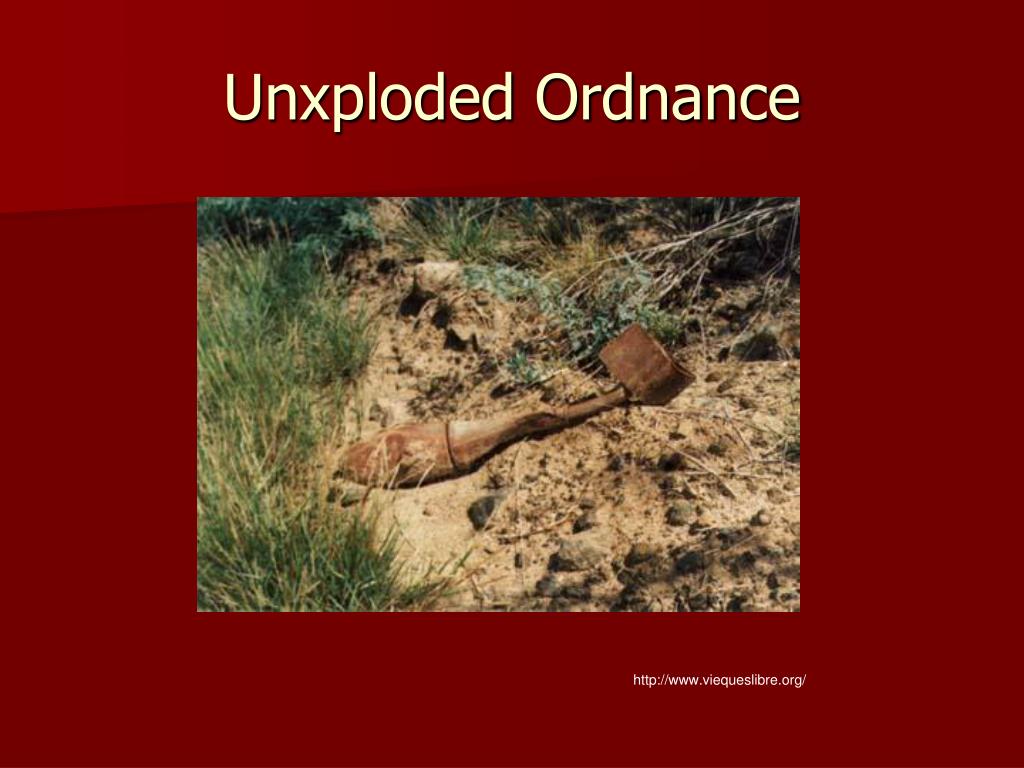The image is a square snapshot of a website with a dark red background and thick red frame. At the top of the frame, in beige lettering with a black drop shadow, it says "unexploded ordnance." The image itself is a rectangular photograph showing a rusty bomb or rocket, around 12 to 15 inches long, lying in a dirt field amidst green grass, dead branches, and gray dirt. The ordnance appears sunken and broken. Below the photograph, the website address is noted in small white lettering: "http://www.viequeslibre.org."